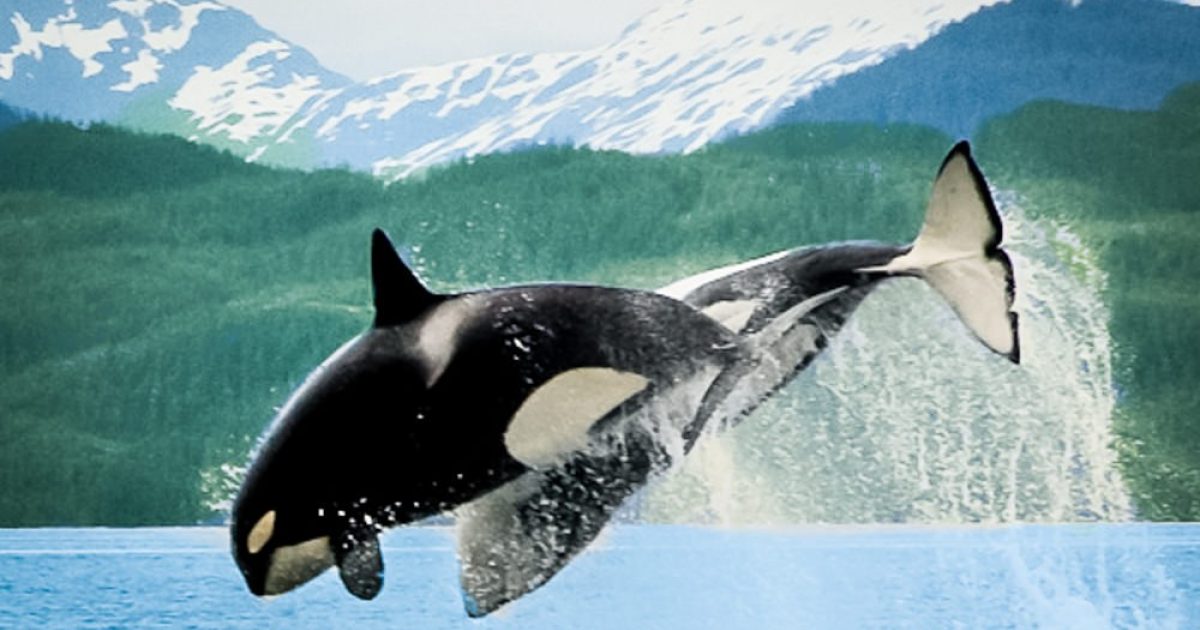This captivating color photograph, oriented in landscape, showcases two majestic killer whales (orcas) leaping out of a medium blue ocean. The orca in the foreground, characterized by its black body and distinctive white markings near its eye and belly, is hunched and facing the bottom left of the image with its tail splashing water to the bottom right. The second whale, slightly behind and higher, appears to have more black and white striping, with its white tail prominently visible, belly facing the viewer, and tail positioned towards the upper right. The scene is set outdoors in daylight under a gray sky, with water droplets and splashes accentuating the dynamic motion of the whales in midair. The serene background features a lush, green hillside dotted with trees and further beyond, a striking snow-capped mountain range, suggesting a location reminiscent of Washington State or Alaska. The image artfully captures the raw beauty and power of nature in a moment of absolute realism.